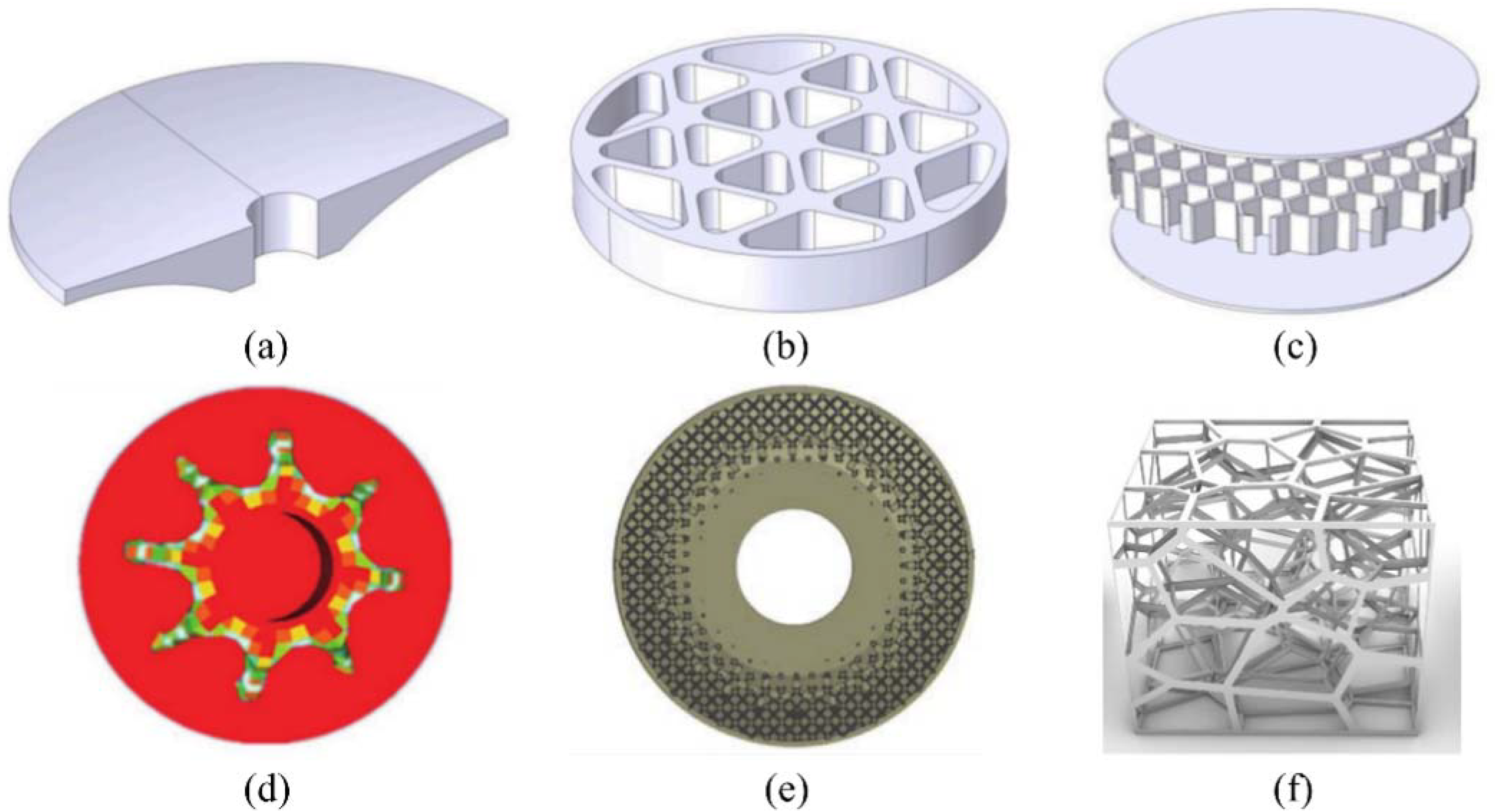The image features six distinct shapes labeled A through F, each varying in form and detail. Starting with A, it is a half oval with a circular cut-out in the middle, potentially for inserting a rod or component. B is designed like a honeycombed circle, featuring a pattern of hexagonal shapes. C resembles a layered cookie (like an Oreo), with concentric darker and lighter gray rings, tapering into a white center, and contains little square elements inside. D stands out as a vibrant red circle superimposed with additional red, green, and white circular shapes, each with small protruding knobs around its perimeter. E is another round shape with shades of gray, progressively lighter towards the center and interspersed with hole-like features. Finally, F is a mesh-like square or box, characterized by intricate, angular wiring or cutouts. The colors and forms suggest they are various parts or components, possibly fitting together in some way, and might be various stands, mounts, or logos.